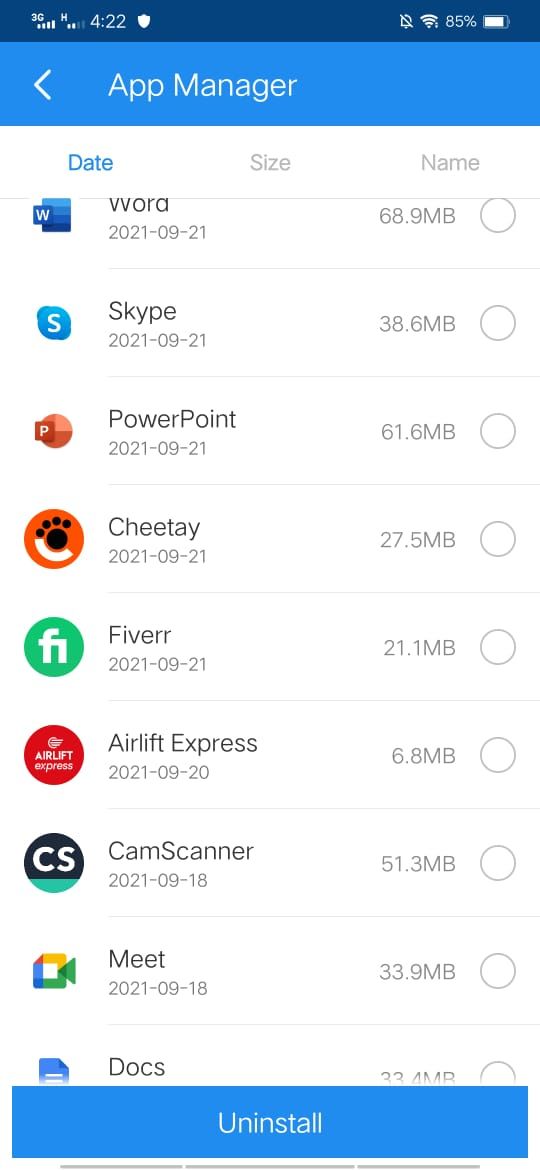The image is a detailed screenshot of a cell phone's "App Manager" interface, highlighting various elements that provide a comprehensive overview of the device's status and installed applications. At the very top of the screenshot, the phone’s status bar can be seen, showing a battery life of 85%, connectivity status indicating a 3G network with four signal bars, and the time displayed as 4:22, though it's unclear whether it’s a.m. or p.m. The background of the status bar is divided into a darker blue for the time and connectivity indicators, reinforcing that this is an older model phone.

The main part of the screenshot prominently features the "App Manager" title just below the status bar, followed by a list of installed applications. Each listed application includes the app name, installation date, and size. Applications visible in the screenshot include Vora (68.9 MB, installed on 9-21-21), Skype, PowerPoint, Cheetah, Fiverr, Airlift Express (6.8 MB, installed on 9-18-21), Meet, and CamScanner, among others. In total, around ten applications can be seen, demonstrating varying sizes and installation dates, helping to provide a snapshot of the phone's usage over time. At the bottom of the list, a button labeled "Uninstall" is present, suggesting that the user can select this to remove any unwanted applications.